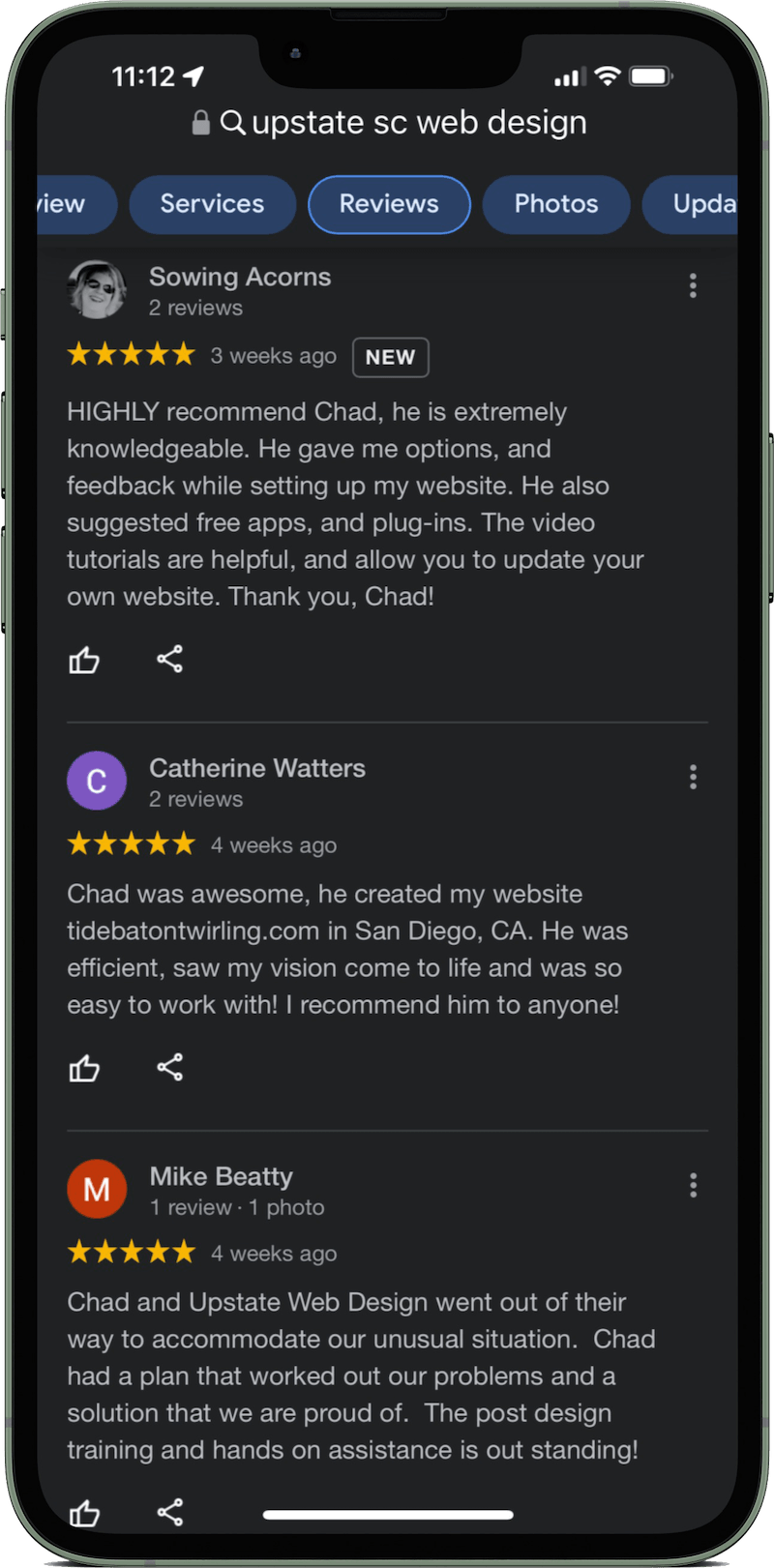A screenshot on a smartphone, showcasing a typical iPhone interface, is displayed. The distinct iPhone format is evident, with a black bar at the center top housing the front camera and speaker. The power button is visible on the right side, while the volume buttons and silent mode switch are on the left. At the bottom, a white bar for switching tabs is present. The top-left corner displays the time, and the top-right corner shows Wi-Fi, battery, and signal indicators.

The page on the phone is in dark mode, with a dark gray background indicating night mode. The screenshot captures a Google search page with the search query "Upstate SC Web Design." The search bar at the top features a lock icon and a search icon. Below the search bar are blue tabs labeled "Overview," "Services," "Reviews," "Photos," and "Updates." The "Reviews" tab is highlighted in blue.

The screenshot further displays three reviews from different users, each rated five stars. Each review includes the user's icon on the left, their name at the top, the rating, the timeframe of the review, and a paragraph detailing their positive experience with an employee named Chad.